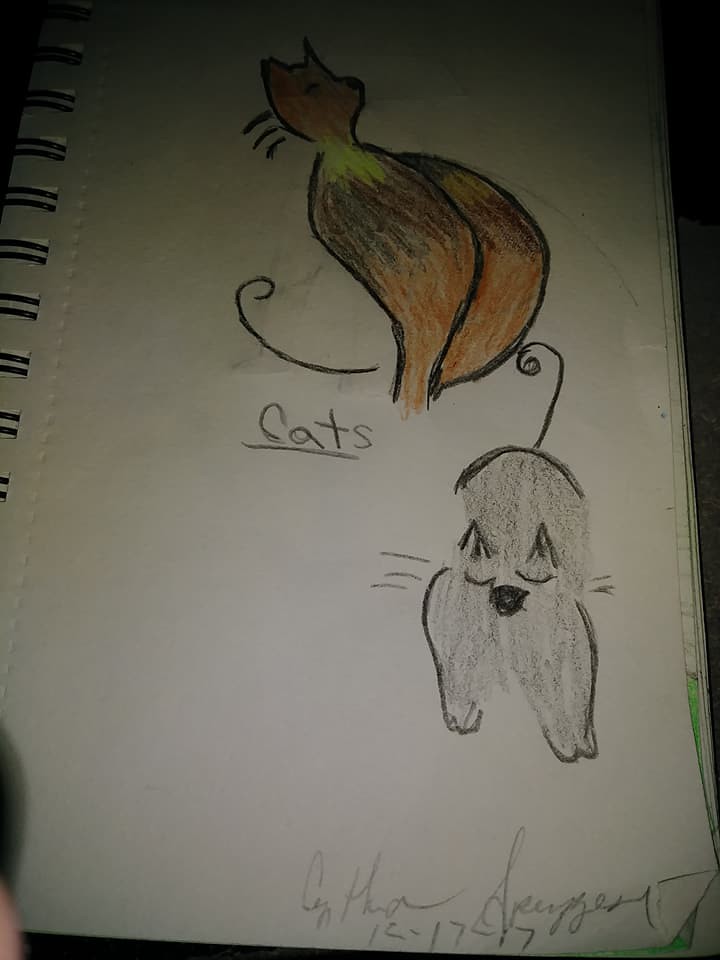This photograph captures hand-drawn images within a sketchbook, set against a background of white, unlined paper. The sketchbook's black spiral binding is visible on the left side of the frame. The artwork features two feline sketches rendered in rich, textured colors. The top cat is illustrated in a palette of orange, yellow, and black hues. It is depicted in a seated position with black whiskers, a black nose, a black eye, and a black tail. Beneath this cat, the word "Cats" is inscribed. 

Below this, a second cat is drawn in varying shades of light and dark gray. This feline appears to be partially lying down with its tail upraised and curled. Its ears are perked up attentively, and it has two eyes, a nose, and delicate whiskers on either side of its face. The cat's paws are extended in a relaxed manner. The lower corner of the sketch features the artist's signature, accompanied by a date, adding a final touch of authenticity to the artwork.